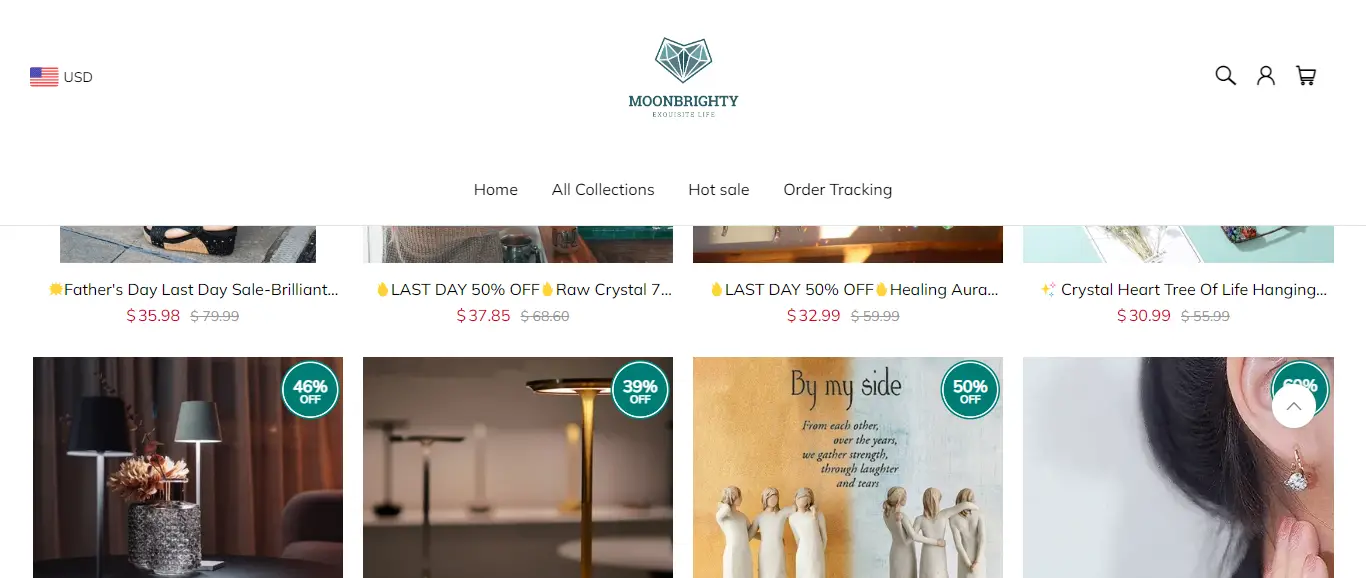Screenshot of Moonbritey E-commerce Website

This detailed screenshot showcases the Moonbritey e-commerce website, which specializes in lifestyle and home decor items. At the top of the page, the header prominently features the website's name, "Moonbritey," accompanied by its logo. The navigation menu includes links to essential sections such as Home, All Collections, Hot Sale, and Order Tracking, along with icons for search, user account, and shopping cart on the right side. In the top-left corner, the currency selector displays the USD currency, indicated by an American flag, suggesting the website’s language and currency settings.

The main section of the screenshot features a collection of product listings under various promotions and discounts. Highlighted offers include:
1. **Father's Day Sale** - "Last Day Brilliant," priced at $35.98, reduced from the original price of $79.99.
2. **Last Day 50% Off Raw Crystal** - Priced at $37.85, reduced from $68.60.
3. **Last Day 50% Off Healing Aura** - Priced at $32.99, reduced from $59.99.
4. **Crystal Heart Tree of Life Hanging** - Priced at $30.99, reduced from $55.99.

Additionally, other products are displayed with varying discount percentages of 46%, 35%, 9%, and 50%. The product images are of high quality, showcasing a variety of items such as lamps, wall art, and jewelry. The website itself is designed with a clean and minimalistic aesthetic, emphasizing product images and discounts to enhance customer focus on the available items.